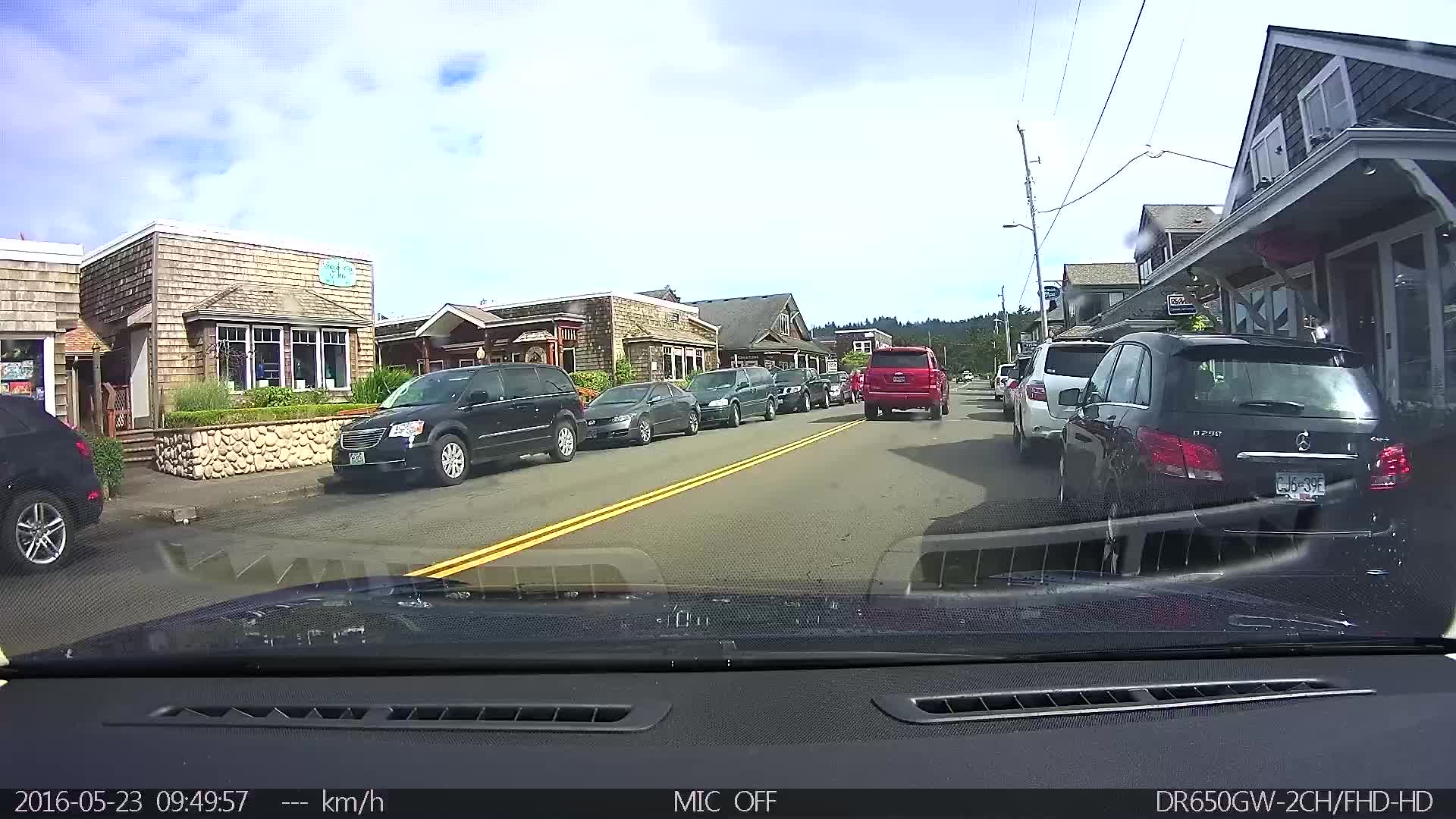The image, taken from the dashboard of a car on May 23, 2016, at 09:49:57 AM, captures a scene through the windshield showing a two-way road with a yellow divider. On the lower right of the image, "DR6550GW-2CH/FHD/HD" is displayed, indicating the dash cam model, and "Mike off" appears in the middle, confirming the microphone status.

The road ahead features multiple vehicles, including a prominent red SUV directly in front. Several cars are parked along both sides of the street. On the left side, there are wooden buildings, including what appears to be a restaurant or store with distinctive wood paneling and old-timey aesthetics. On the right side, a telephone pole with wires stretches into the distance, accompanied by trees and a distant hill covered in foliage. The sky is partly cloudy, enhancing the clear day ambiance, as the car moves through what appears to be a quaint town setting with various retail establishments lining the street.